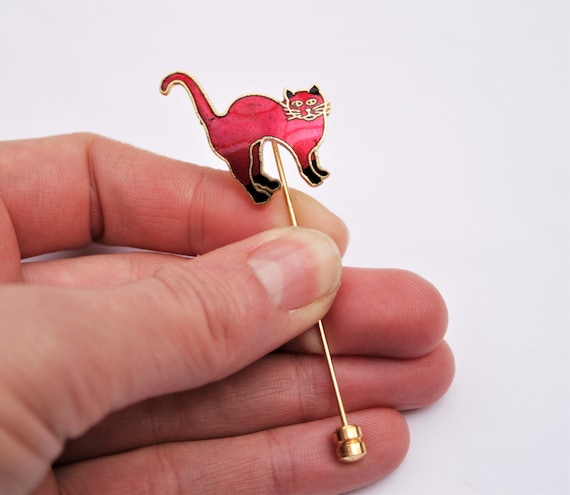This close-up photograph captures a person's hand, with their thumb and index finger delicately holding a small, gold ornament. The ornament is a pin featuring a vividly colored, pinkish-red cat. This tiny cat, which is no bigger than the fingertip, has an arched back, suggesting a humped posture, and it prominently displays gold outlines around its body, paws, legs, tail, face, and whiskers. The cat sports black ears and paws, with its whiskers also rendered in gold. The fine details of the cat’s face, including its black eyes, are clearly visible, emphasized by the gold outlines. The ornament rests partially on the person’s pinky, and the background of the image is a plain white, allowing the vibrant colors of the pin to stand out distinctly.